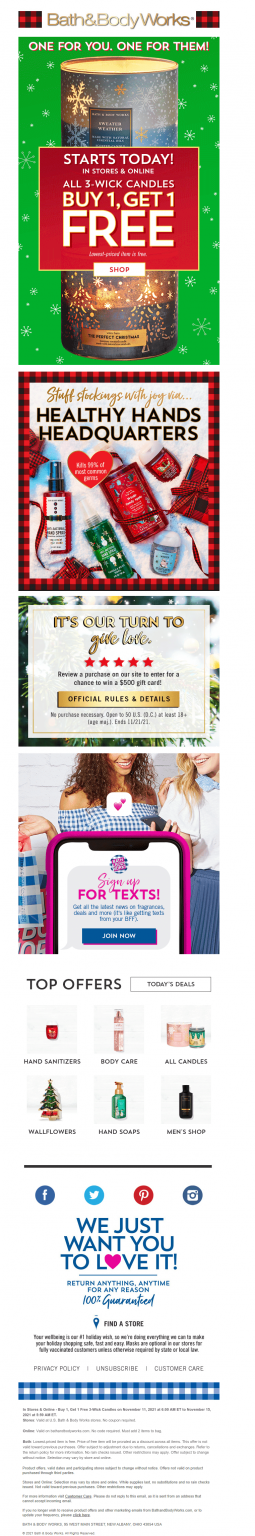Here's a cleaned-up and detailed caption for the image described:

"Online advertisement for Bath & Body Works on a white background featuring several promotional offers and categories. At the top, the Bath & Body Works logo is displayed. Below, a red banner announces 'One for you, one for them' with the text 'Starts today' and 'All 3-wick candles, buy one get one free.' A candle is set against a festive green background with white snowflakes. Further down, a section titled 'Healthy Hands Headquarters' showcases various hand care products. Above this, a black-and-white striped banner reads 'Stuff Stockings with Joy' with some unreadable text. The ad also features a gold hyperlink titled 'Official Rules and Details' suggesting a charity initiative, accompanied by a background with tree graphics. A picture of a smartphone with a pink case promotes signing up for text alerts with the text 'Sign up for Texts' in pink, immediately followed by a blue button with 'Join Today.' The section 'Top Offers' in black highlights categories such as 'Hand Sanitizers,' 'Body Care,' 'All Candles,' 'Wallflowers,' 'Hand Soaps,' and 'Men's Shop,' each with corresponding icons. The bottom of the ad contains legal information."